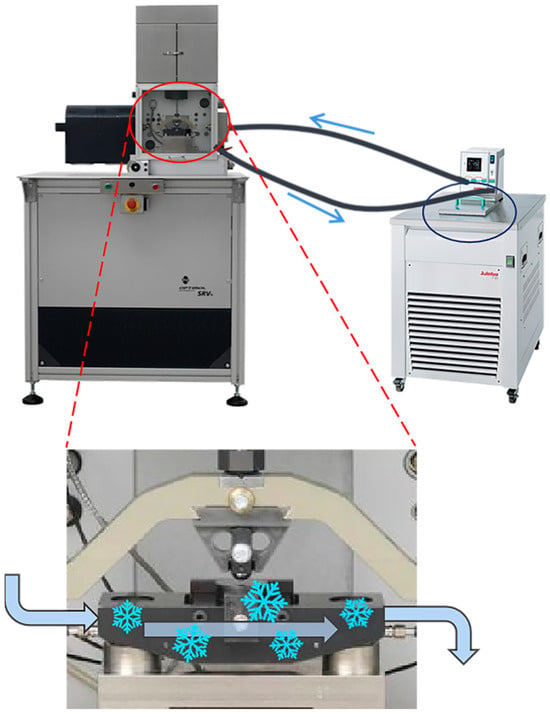The image depicts a detailed, textbook-like diagram of machinery, emphasizing various components and their functions. Centered are three rectangular, cabinet-shaped machines: one on the top left is smaller and gray, and another on the middle right is larger and beige. Each cabinet houses mechanisms on top, connected by black tubes. A marked red oval and dotted red lines focus attention on an area of the gray machine, illustrating its internal workings. Below it, a close-up view gives an inside look of the machine, with blue arrows and bright blue snowflake symbols indicating airflow and cooling processes. The diagram effectively uses lines and colors to explain the machinery's functionality and structure.